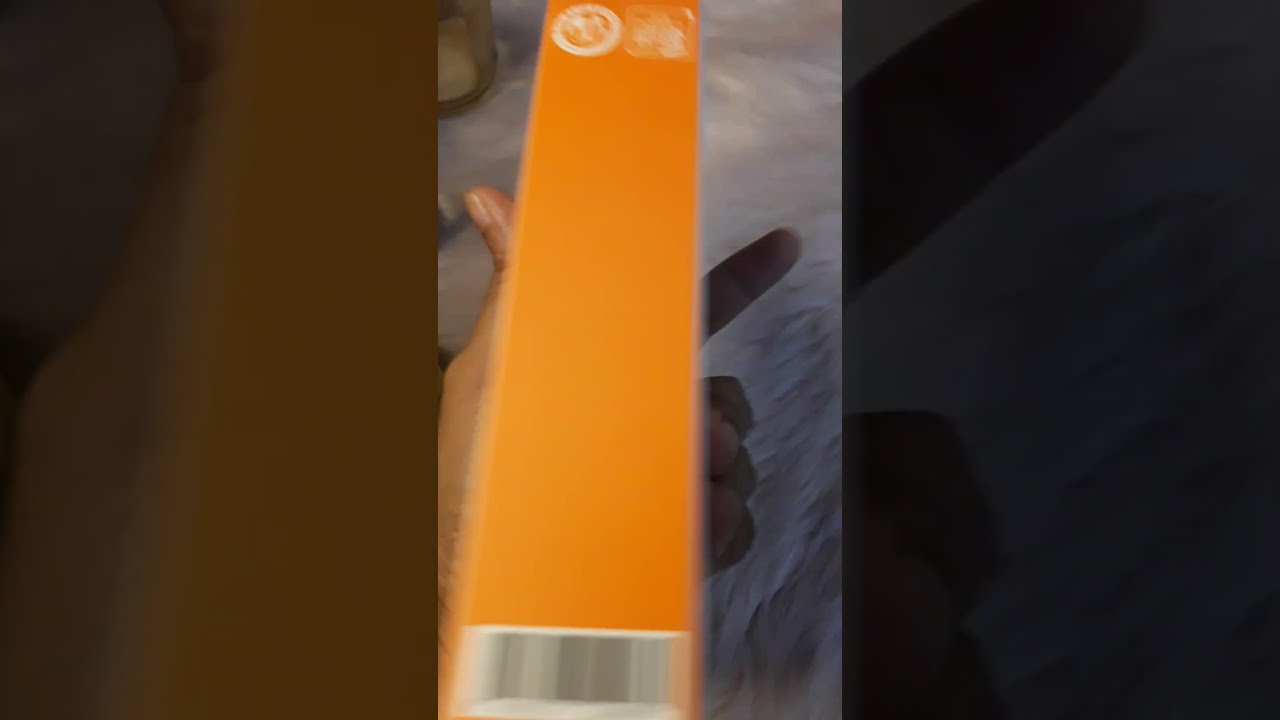The image appears to be a screen grab from an unboxing video, capturing a hand holding a yellow rectangular box with a barcode at the bottom and a faint icon at the top. The hand is positioned palm-up with the thumb slightly bent outward, suggesting a grip on the object. The box appears blurry due to motion, and the scene is set against a white, possibly wrinkled, background, likely a tablecloth or bedspread. The image contains three sections: a well-lit center where the hand and box are most visible, and darker, zoomed-in segments on the left and right showing parts of the hand and shadows. Despite the fuzziness, the overall impression is of an unboxing process, though specific details about the box and background remain unclear.